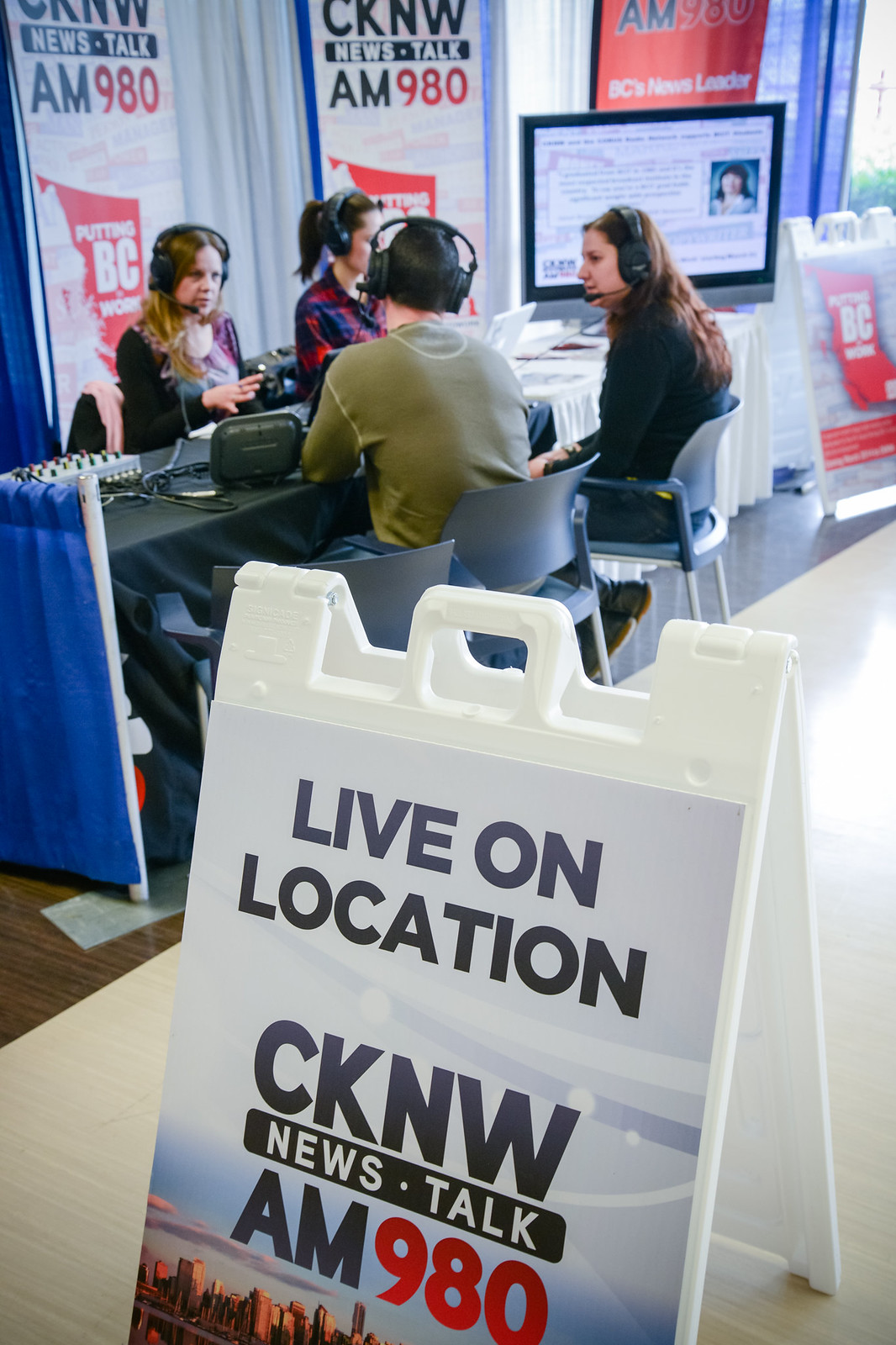In the image, four individuals are seated at a table engaged in a live radio broadcast for CKNW News Talk AM 980. Each person is equipped with headphones and microphones, suggesting they are actively participating in the discussion. A prominent white A-framed sign at the forefront reads "Live on Location CKNW News Talk AM 980" with additional details in white, black, blue, and red text, along with a subtle city skyline at the bottom edge. The table is covered with a gray tablecloth and a white half curtain, adorned with various pieces of electrical equipment. The participants are casually dressed: the man on the left wears a green shirt, the woman next to him sports a blue shirt, the woman opposite her has on a plaid shirt and wears her brown hair in a ponytail, and the woman next to her dons a purplish shirt, her hair long. They are seated on blue chairs, with additional signage in the background that includes white banners labeled "CKNW News Talk AM 980" and a red banner with "AM 980" in blue and yellow letters. The setting appears relaxed yet professional, reflecting a behind-the-scenes moment from a live radio broadcast.